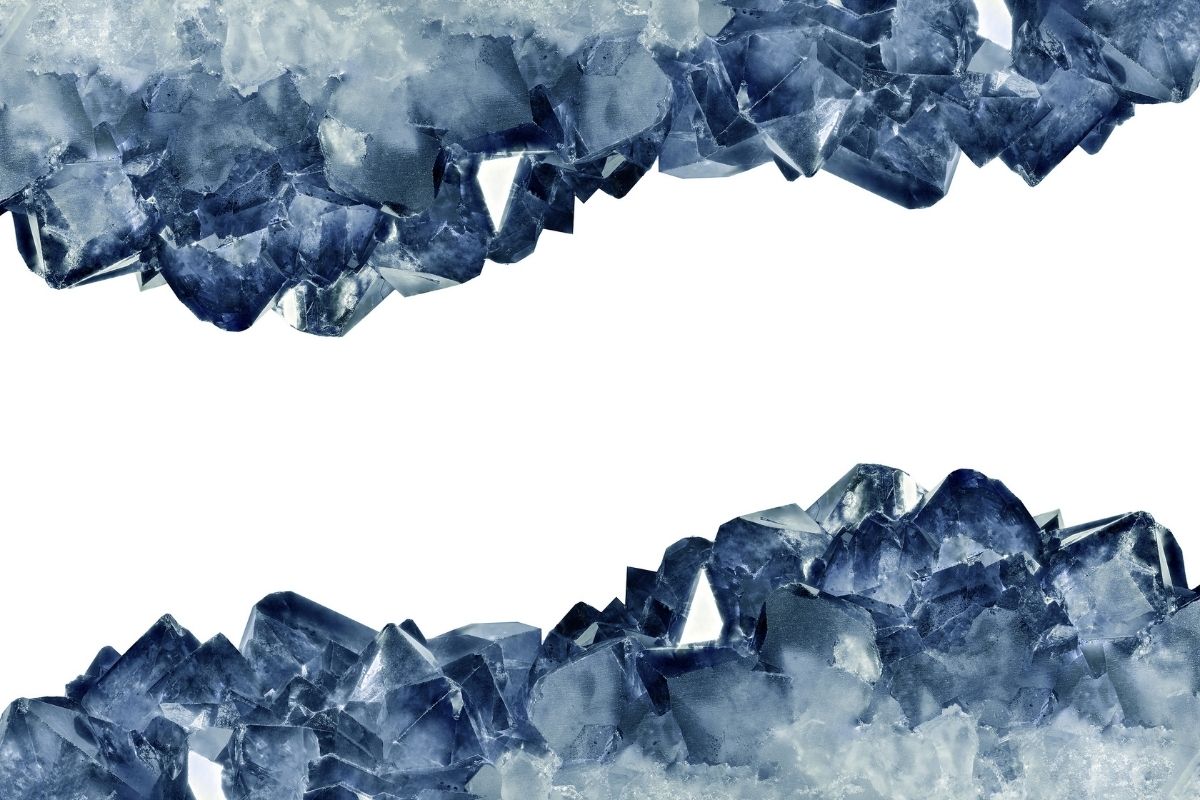This image features a close-up of a striking crystal or mineral structure set against a stark white background. The composition is intriguingly divided, with clusters of crystals at both the top and bottom edges creating a chasm of blank white space in the center. The dominant colors of the crystals are a deep, dark blue and clear to opaque white, giving a glassy, almost mirrored appearance between the top and bottom sections. These crystalline formations predominantly consist of small, angular shapes like cubes and triangles, clustered together on a bigger, less detailed mass. The jagged silhouettes of these rocks render a jaggy, uneven edge both at the top and bottom, enhancing the structure's intricate and rugged aesthetic. The light subtly glistens off various facets, highlighting the fused and sometimes rough textures amid the predominantly angular shapes. The size of the individual crystal facets is roughly around the size of a thumbtip, contributing to the overall detailed and intricate nature of the photograph.